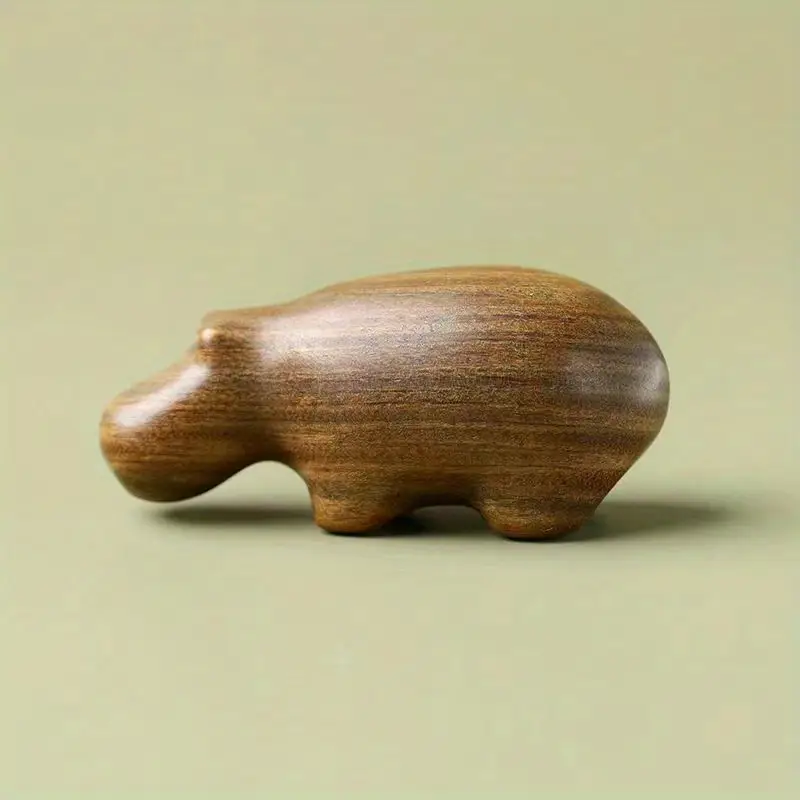The image depicts a simple, abstract wooden figure of a hippopotamus, carved from a medium brown wood with varying shades of light and dark brown wood grain. The wooden hippo is smoothly polished, reflecting light and other objects in the room, especially noticeable around its head and rounded back. Despite its lack of fine detail, the carving hints at the hippo's distinct features such as a large, rounded snout, possibly indicated eyes, and four stumpy legs. The side view of the figure reveals one roughly carved ear and a large, cylindrical nose and mouth. The figure casts a shadow on an olive green surface in a well-lit area, with the background appearing grayish pink. The hippo figure, which could be roughly hand-sized, exudes a decorative charm despite its simplistic and abstract representation.